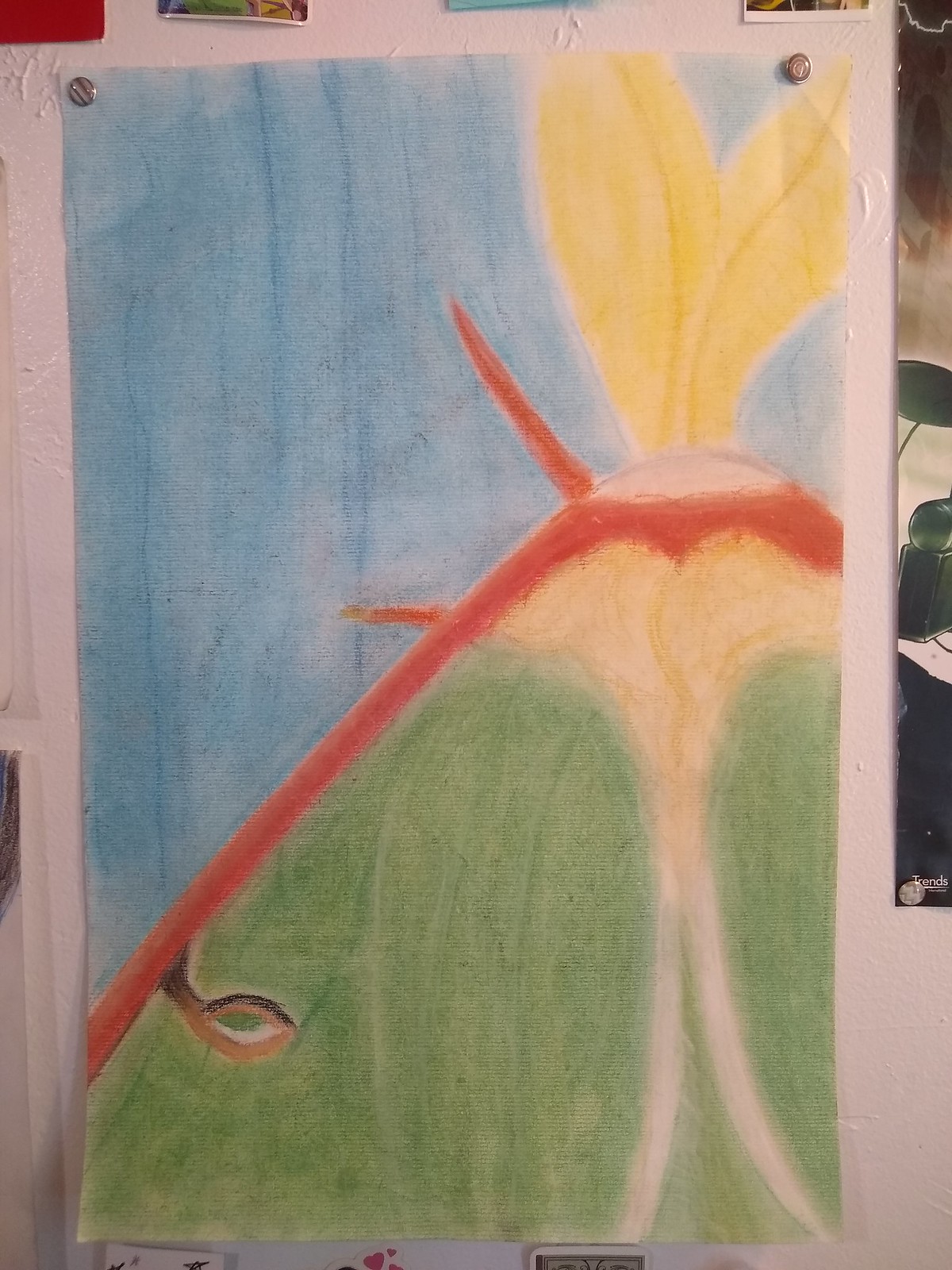This is a vibrant, color photograph of an abstract drawing prominently displayed on a wall. The artwork, which could have been created by a child or as an artistic rendering, dominates the frame. On the right side of the drawing, there are two bright yellow feathers intricately connected to what resembles an onion bulb. Extending from this bulb are two stalks, adding a sense of organic fluidity to the composition. Additionally, a red line emerges from the bulb, running diagonally towards the lower left-hand corner of the drawing, creating a dynamic visual element. The background of the piece is filled with rich green hues, while the top left-hand corner transitions into a serene sky blue, offering a striking contrast. The overall effect is a captivating blend of colors and shapes, evoking both simplicity and complexity.